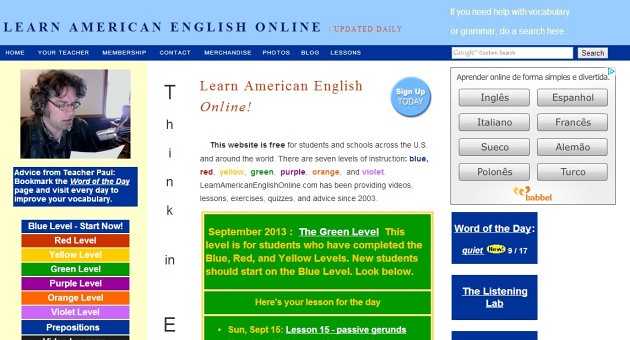This detailed screenshot showcases a website dedicated to teaching American English online. At the very top, a light blue horizontal bar features the phrase "Learn American English Online" in dark blue, capital letters, accompanied by an orange "Updated Daily" notification. Just below, in light yellow text, it suggests, "If you need help with vocabulary or grammar, do a search here," followed by a search bar for easy navigation.

Prominently displayed in the center is the main message, "Learn American English Online!", emphasized in vibrant orange font. The website's navigation bar includes categories like Home, Your Teacher, Membership, Contact, Merchandise, Photos, Blog, and Lessons.

To the left is an organized column listing different proficiency levels, each marked by distinct colors: Blue, Red, Yellow, Green, Purple, Orange, and Violet, with an additional section for Prepositions. Each level invites users to "Start Now" and progress through the structured curriculum. An image of a man wearing glasses, presumably Teacher Paul, is also visible with a note encouraging users to bookmark the "Word of the Day" page for daily vocabulary improvement.

Additionally, multilingual buttons are displayed, providing translation options for various languages such as Italiano, Sueco, Polonese, Turco, Francés, and Espanhol (E-S-P-A-N-H-O-L). A bold blue circular button labeled "Sign Up Today" in white text offers an easy way for visitors to join the learning platform. The overall layout is set against a clean white background, enhancing readability and user engagement.